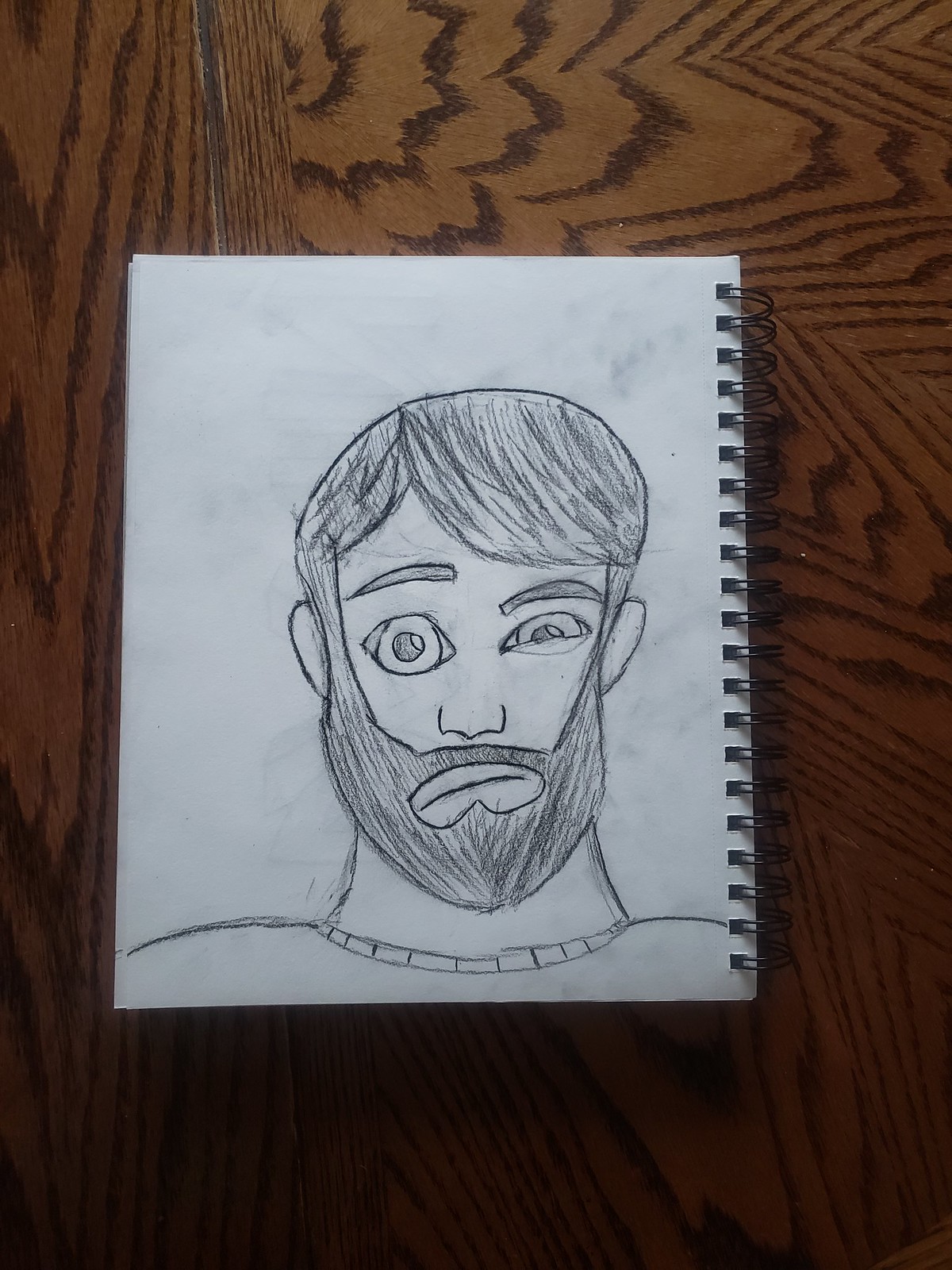The image features a detailed sketch centered on a spiral-bound sketch pad, which is placed on a brown, wood-grained table. The pad's spiral binding is positioned on the right side. The sketch depicts a man with dark hair and long sideburns that extend into a beard and mustache. One of his eyes is wide open while the other is partially closed, and he sports a cocked grin. He is dressed in a simple, close-neck shirt. The drawing is primarily composed of clean lines, with some shading used to give depth to the hair, beard, and mustache.